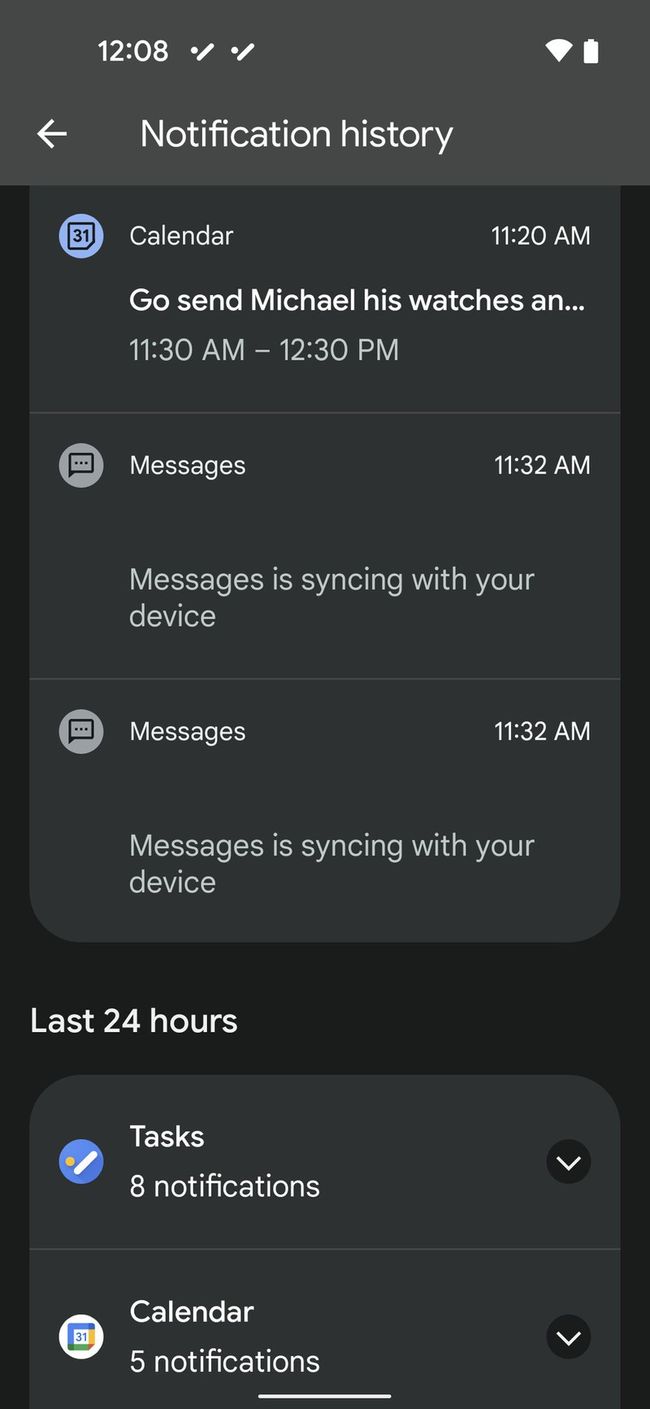Here is a detailed and cleaned-up caption for the image you described:

---

The image is a screenshot of an app's history tab. At the top left corner, the time displayed is 12:08, indicative of when the screenshot was taken. On the top right corner, the WiFi icon and battery icon are visible.

The main title reads “Notification History.” The first entry under this title is from the Calendar app, timestamped at 11:20 AM. The visible part of the notification reads: “Go send Michael his watches,” and the rest of the text is cut off. Another entry from the Calendar shows a scheduled event from 11:30 AM to 12:30 PM.

Below the Calendar entries, there are two identical notifications from the Messages app, both timestamped at 11:32 AM and each stating: “Messages is syncing with your device.”

A header titled "Last 24 hours" follows. Under this, the first entry shows “Tasks” with 8 notifications, accompanied by a down arrow on the right side. The next entry is from the Calendar, showing 5 notifications, also accompanied by a down arrow on the right.

---

This cleaned-up caption provides a more structured and detailed description of the image contents.